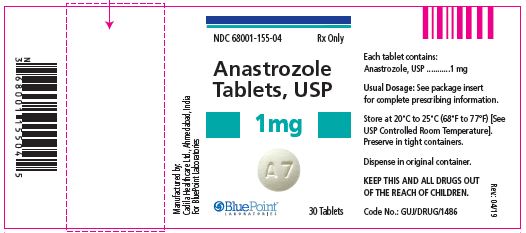The image depicts a medication label styled as a horizontal white rectangle. On the left side, there is a black barcode, and the entire label is outlined in red. Adjacent to the barcode, extending horizontally, there is a band enclosed by a red dotted line, leading to the main area of the label. A red arrow points from the left band towards the blank white space in the center.

The central section of the label features a blue band on top, with a green band directly below it. The text in this area is predominantly in black, stating "DNC 68001-155-04 RX ONLY." The medication name "ANZIROTOL ANASTROZOLE TABLETS, USP" is printed in the largest font size on the label, also in black. Next to this, there is a teal-colored box containing the dosage strength, "1MG." This text size matches that of the medication name. On the opposite side of the label, there is another teal box with "1MG" printed in teal.

Below this text, there is a photograph of the actual pill, which is white and imprinted with "AZ." Directly beneath the pill image, the label reads "Blue Point" and "30 Tablets." On the far left side of the label, additional manufacturing information is provided, stating: "Manufactured by CADILA Healthcare Ltd, Ahmedabad, India for Blue Point Laboratories."